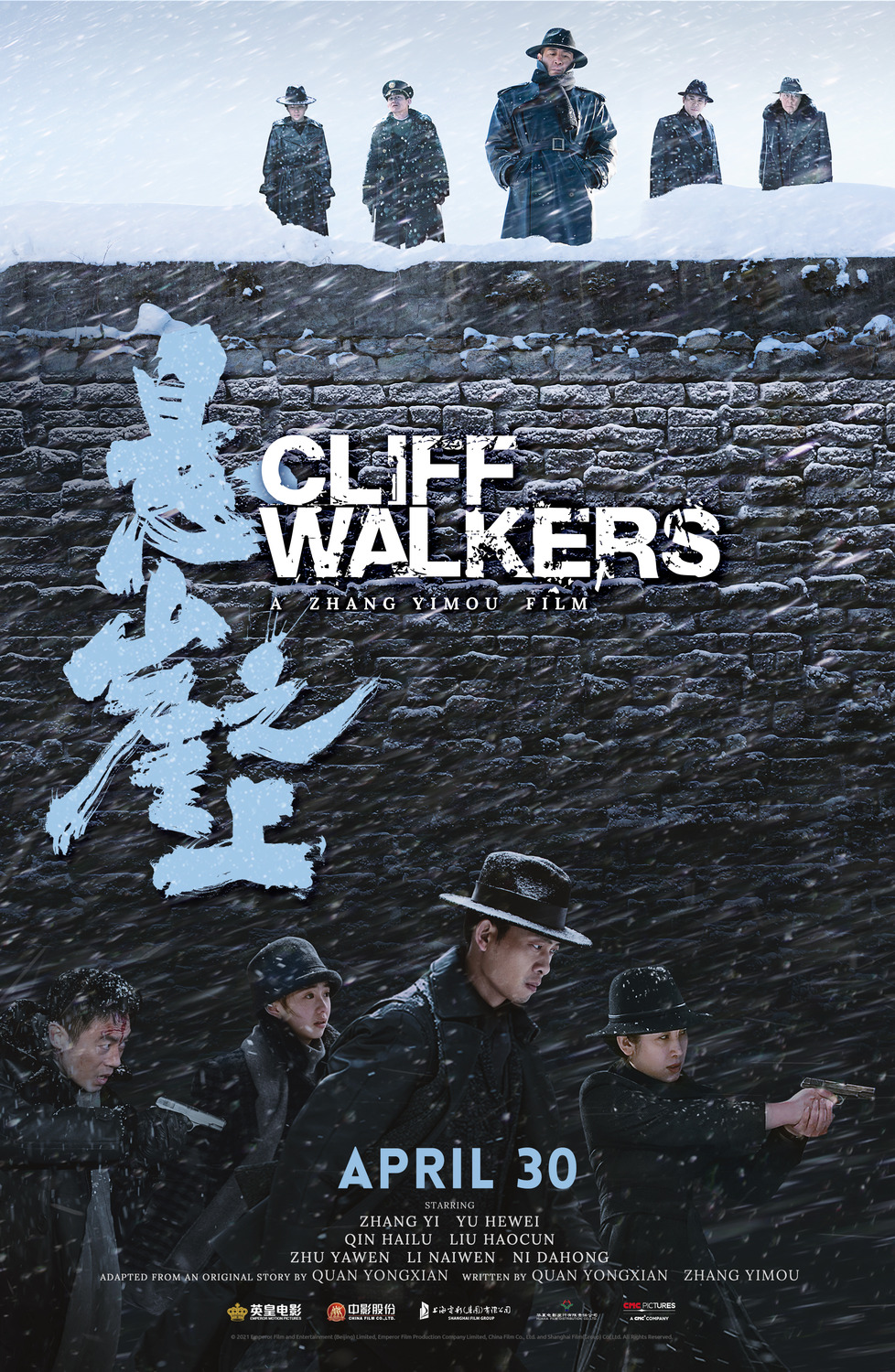This poster advertises the movie "Cliffwalkers," a Zhang Yimou film. The top of the poster features a dark gray brick wall with a layer of snow on its edge. Five figures dressed in black trench coats and black hats peer over the wall. At the base of the wall, four similarly dressed figures stand. On the right, two of them point guns towards the distance, while a figure with short black hair stands on the left, and another man in a black hat looks downward dramatically in the center. The top third of the poster contains the title "Cliffwalkers" in large white text, accompanied by light blue Asian characters and a scattering of white snowflakes. The bottom section provides a release date of April 30 in blue text, followed by a white text listing cast members, including Zhang Yi, Yu Hewei, Qin Hailu, Liu Haokun, Zhu Yaowen, Li Naiwen, Ni Dehong, and the original story's adaptation and writing credits to Kuan-Yong Shan and Zhang Yimou. Several small, unreadable logos cluster at the very bottom. The poster predominantly uses black, gray, and blue tones.